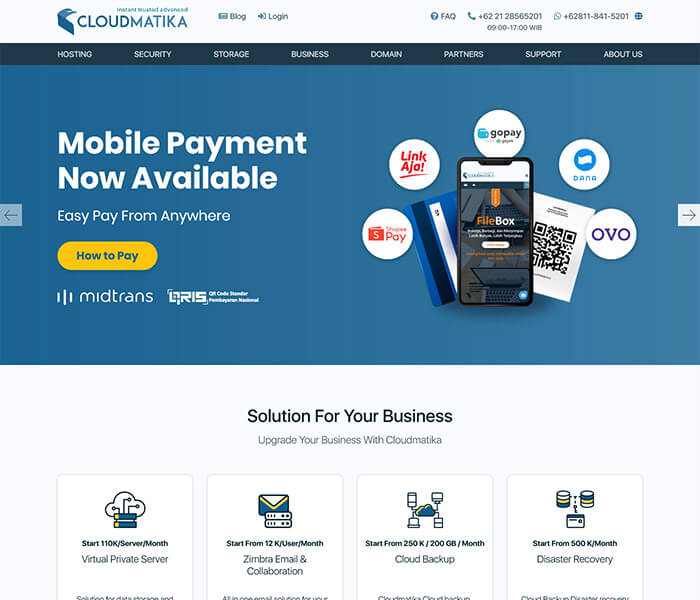The image features a website with a clean, structured layout. At the very top, a white border displays the text "Cloud Matica" in dark blue, with a logo situated to the left. To the right of this text, there are navigation links labeled "Blog," "Login," and "FAQ." Further to the right, a phone icon with the number "+62 21 28 56 5201" is visible.

Beneath this section, a black horizontal menu provides clickable links labeled "Hosting," "Security," "Storage," "Business," "Domain," "Partner," "Support," and "About Us."

The main body of the webpage has a dark blue background, with large white text proclaiming, "Mobile Payment Now Available." Smaller text underneath reads, "Easy pay from anywhere." Centrally placed below this is an oblong yellow button with dark blue text that says, "How to Pay."

Finally, beneath the button, the text "Mid Trends" appears. To the right of this text, there is an image of a smartphone. Above the smartphone, circles displaying different brand names, including "OVO," can be seen.